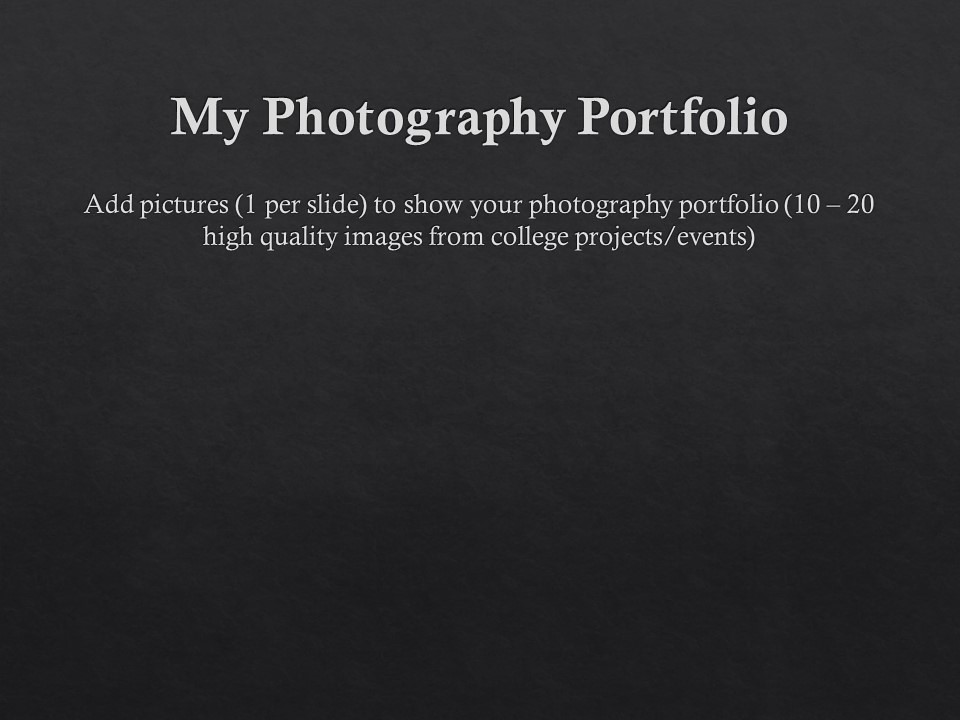This image presents a simplistic design with a predominantly black background that transitions to gray near the top. It resembles a scanned or printed piece of paper. Centrally located at the top of the image, bold white text reads "My Photography Portfolio," using capital letters for emphasis. Below this, there are two indented lines of white text: "Add Pictures (one per slide) to show your photography portfolio (10-20 high-quality images from college projects/events)." The image is slightly wider than tall, and there are no additional footers, headers, or borders, contributing to its straightforward, monochromatic aesthetic.